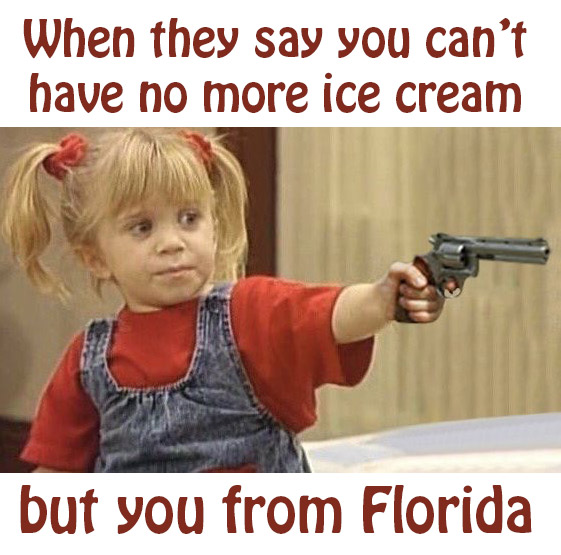A humorous internet meme features Michelle from Full House, portrayed by Mary-Kate and Ashley Olsen, holding a silver toy revolver with a wooden handle in her left hand. Michelle, who sports blonde pigtails tied with red scrunchies, wears a red shirt under denim overalls. She stands indoors against a cream-colored wall with a dark wooden beam visible in the background, and only the upper half of her body is shown. Her expression is neutral, tinged with slight discontent. The meme text, in maroon-colored lettering, reads at the top: "When they say you can't have no more ice cream," while the bottom text continues: "but you from Florida." The text is positioned above and below the centered image, all set against a white background.